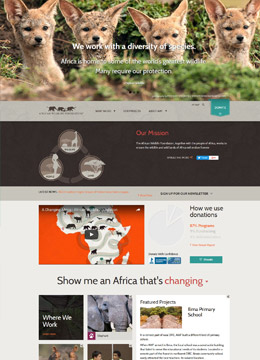In this image, the top center features four foxes with light brown fur, dark eyes, and noses. The inside of their ears is lighter, almost white. The foxes are seated in a green grassy field. Below them, there are three circles, each bearing a different animal logo. On the right side of the image, the phrase "OUR MISSION" is displayed in red text.

The bottom half of the image contains a squared box with a video thumbnail. The video is not playing, but the thumbnail shows an orange background with a white shape that features multiple small animal logos. Below this, the text reads, "Show me an Africa that's changing." To the bottom left of the image, there are four photos depicting an elephant and several humans, accompanied by the text "Where we work."

On the bottom right, there is a small article. Adjacent to it, towards the middle right of the image, is a section titled "How we use donations," followed by a detailed description.